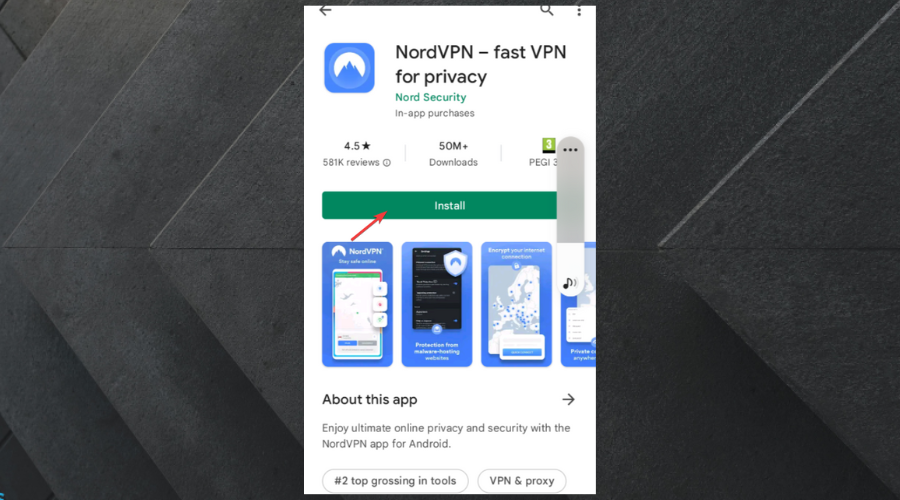The image is an advertisement for the NordVPN virtual private network service. The background consists of grey tiles arranged almost like petals of a parapet flower, giving the image a structured and sophisticated look. In the foreground, a clean, white rectangle prominently displays the NordVPN logo along with the taglines "Fast VPN for privacy" and "Nord Security," highlighted in green. Below this, it states that in-app purchases are available. 

The advertisement proudly shows a high user rating of 4.5 stars based on 581,000 reviews and notes that the app has been downloaded over 50 million times. At the center of the image, a green rectangle with the word "Install" written in white invites users to download the app, further emphasized by a red arrow pointing towards the install button.

Beneath this call-to-action are several small images, representing the various features of NordVPN, although their size makes it difficult to discern specific details. The first image is in color, the second is in black and white, and the third appears to be a map, suggesting functionality related to geographic security measures.

At the bottom of the advertisement, there is a section labeled "About this app," which can be expanded for more detailed information about NordVPN.